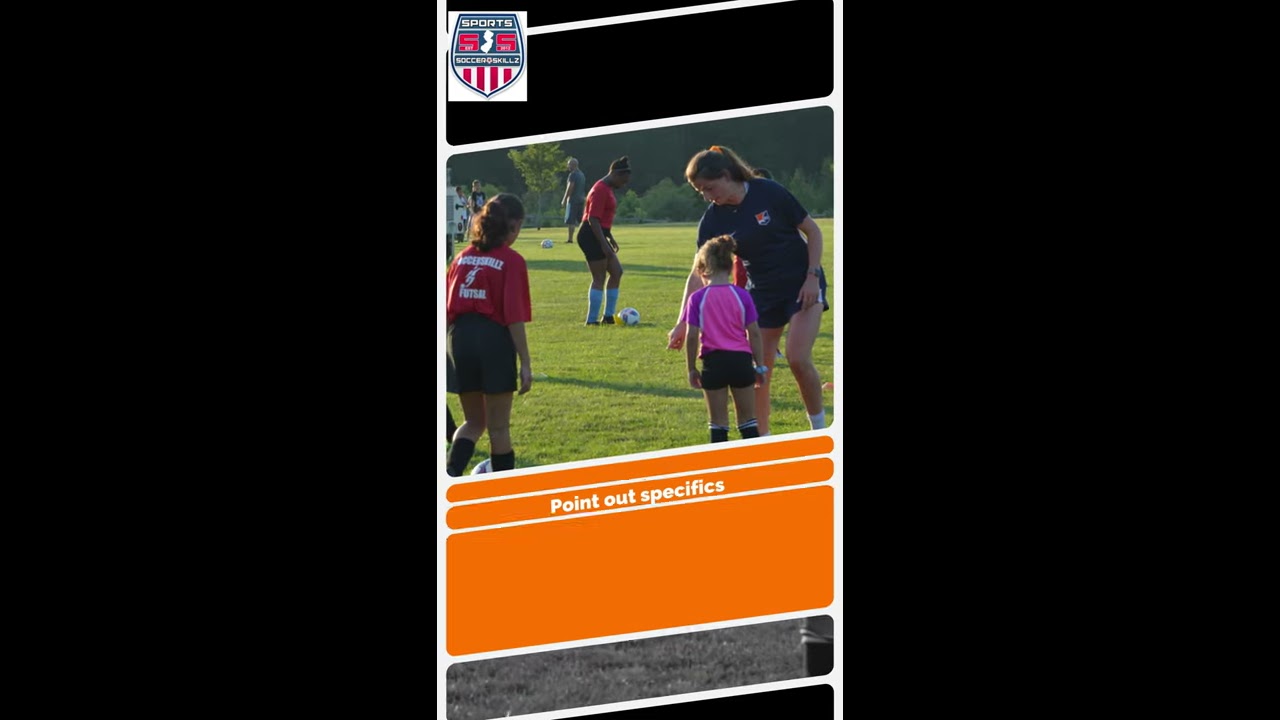The image, taken in portrait mode, features a colorful and dynamic scene of a soccer training session designed for an informational advertisement. At the top, there is a black bar angled upwards, alongside a white square with a blue-outlined shield showcasing the word “sports” in white. Just beneath the word "sports," there are two indistinct characters that appear to be either "S" or "5", and lower down the shield, four red bars are displayed vertically.

Dominating the center of the image is a vibrant outdoor photograph on a lush green soccer field. A young girl in a pink and purple shirt with black shorts and soccer socks stands to the right with her back to the camera. An older woman in a black t-shirt and black shorts is beside her, seemingly providing guidance. To the left, two individuals are visible in red tops and black shorts, with one having her back to the camera showcasing some hard-to-read white lettering.

At the bottom of the photo, three orange diagonal stripes appear, one of which contains the white text “point out specifics.” Overall, the image captures a lively moment of hands-on soccer coaching, emphasizing instructional methods for engaging young players in the sport.